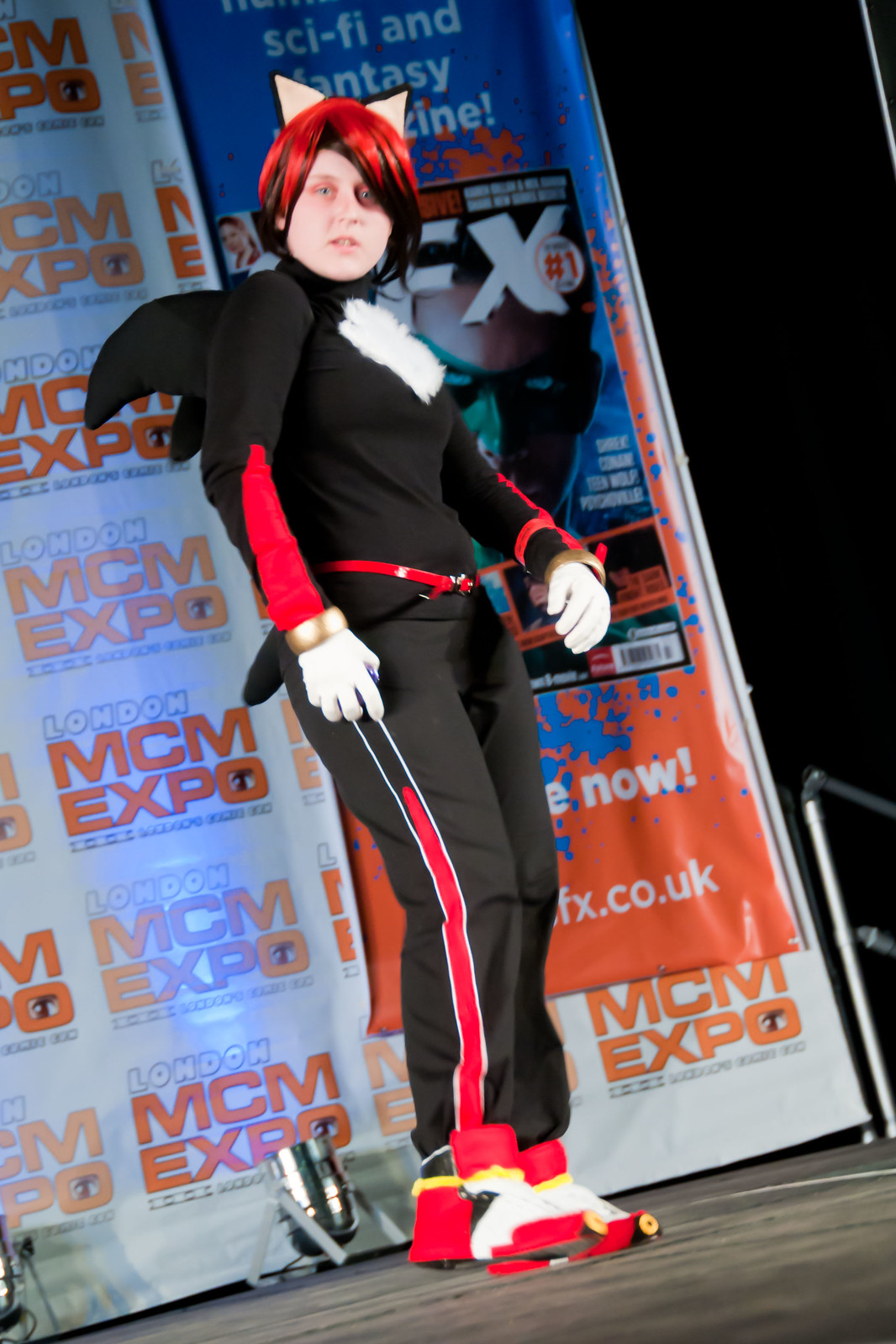The image depicts a woman in a detailed cat-themed costume, likely cosplaying as a video game character, standing on a stage at the London MCM Expo. She has short, red and black hair with two triangular yellow cat ears. Her outfit is predominantly black with a long-sleeved turtleneck top and matching pants. The top features white fur on the chest and red stripes on the forearms, complemented by gold rings on her wrists and white gloves on her hands. The pants have a distinctive red stripe bordered by white lines running down the sides. She is also wearing a red belt with a silver buckle and red high-top sneakers with white stripes and laces. Her ensemble is completed with black wings and a tail. The background prominently features a repeatedly printed "London MCM Expo" banner. Additionally, there is a silver railing visible in the corner of the stage, and the woman is looking straight at the camera.